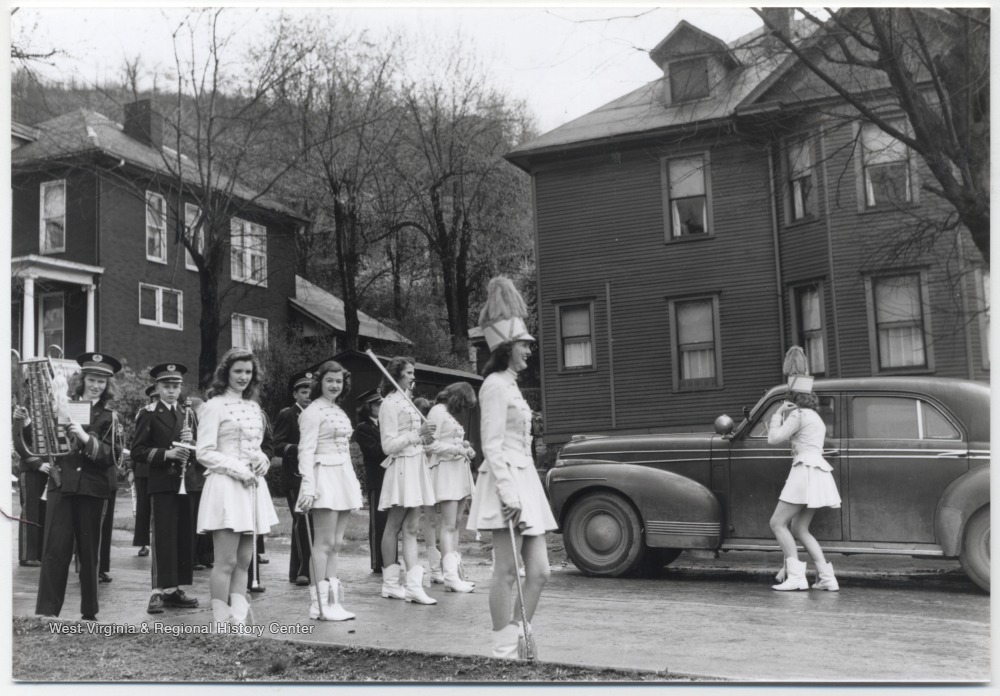This black-and-white photograph, likely from the 1940s, captures a street scene featuring a marching band and its accompanying majorettes. In the forefront, a line of white women, dressed in matching uniforms consisting of very short white miniskirts, long-sleeved tops, and white boots, are standing poised with batons in hand, suggesting they are drum majorettes or baton twirlers. The lead majorette, distinguished by a hat adorned with a large feather plume, stands at the front, while another leader appears to be engaged near an older vehicle—possibly a car from the 1920s to 1940s—seen towards the right in the background. Behind the majorettes, a band dressed in black uniforms with matching caps can be seen holding various instruments, such as clarinets, with two houses visible further back. The image is labeled with "West Virginia and Regional History Center." The camera angle provides a side view, allowing a glimpse of the organized alignment of the participants on the street.